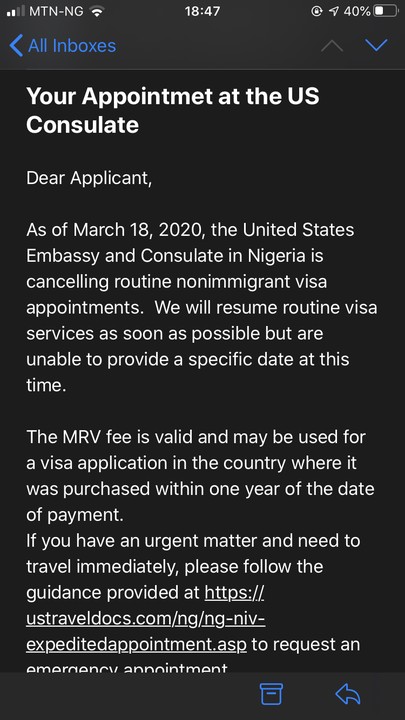### Descriptive Caption for Screenshot

The screenshot appears to be from a smartphone or tablet, showcasing various notifications and interface elements. Here’s a detailed breakdown:

#### Top-Left Corner Interface
- **Cellular Signal**: Two out of four bars indicate moderate network strength.
- **Carrier Information**: Displays "MTN - NG," referring to MTN Nigeria.
- **Wi-Fi Signal**: Two out of three bands are active, indicating a decent Wi-Fi connection.
- **Time**: The device shows 18:47 in military time, displayed in white text.
- **Security and Battery Icons**:
  - A white circle with a lock indicates the device is secured.
  - An arrow pointing to the right followed by "40%" next to a battery symbol shows the current battery level.

#### Email Interface
- **Navigation and Status Icons**:
  - A dark blue icon with a rising arrow points to "All Inboxes."
  - A gray arrow pointing up and a blue arrow pointing down appear on the right, likely indicating actions for sorting or filtering emails.
  
- **Message Content**:
  - **Header**: Bold white text reads, “Your appointment at the US Consulate.”
  - **Body**:
    - Regular white text continues with, “Dear Applicant, as of March 18th, 2020, the United States Embassy and the Consulate in Nigeria are canceling routine non-immigrant visa appointments. We will resume routine visa services as soon as possible but are unable to provide a specific date at this time.”
    - **Additional Information**:
      - Bold text states, “The MRV fee is valid and may be used for a visa application in the country where it was purchased within one year of the date of payment.”
    - **Urgent Travel Guidance**:
      - The text advises, “If you have an urgent matter and need to travel immediately, please follow the guidance provided at” followed by a URL.

- **URL**: The specific web address for requesting an emergency appointment is:
  `https://ustraveldocs.com/ng/ng-niv-expeditedappointment.asp`

- **Email Actions**:
  - A blue trash can icon indicates the option to delete the email.
  - A blue upward-triangle icon, likely for archiving or marking the email. 

This caption provides a comprehensive description of the screenshot, highlighting key interface elements and the detailed content of an email concerning visa appointments at the US consulate in Nigeria.